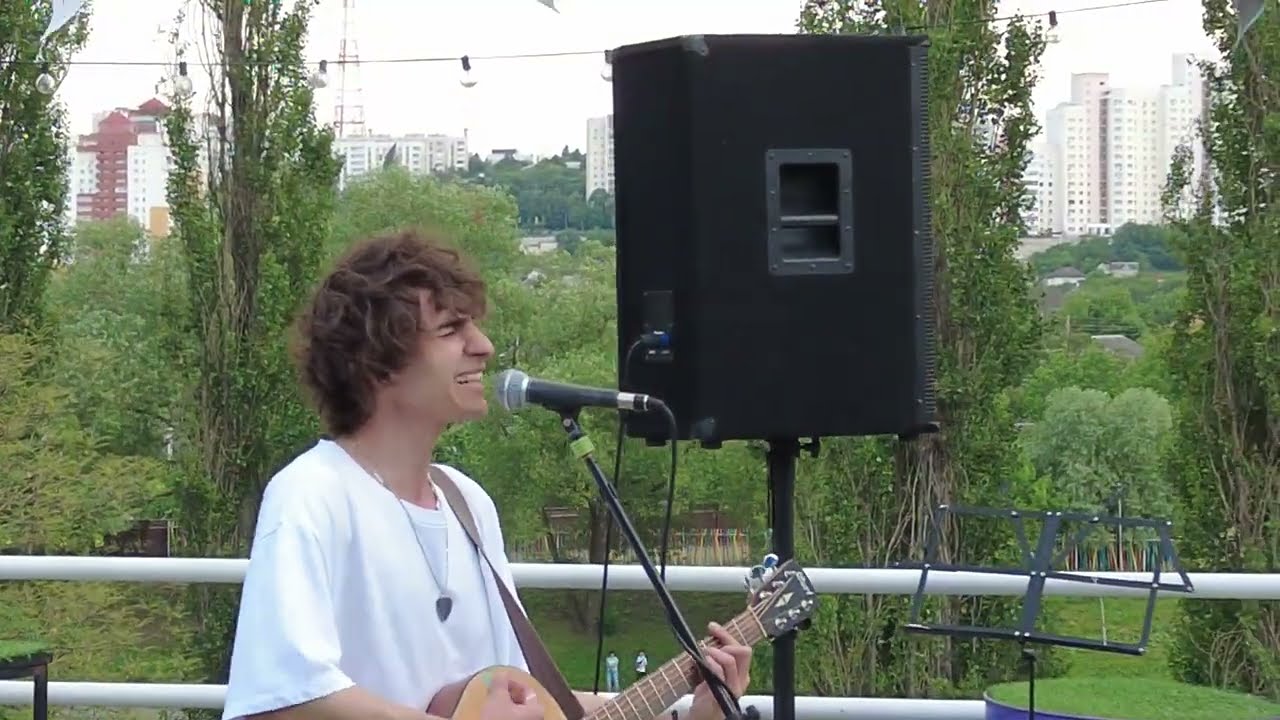In this photograph, a man with long, brown, slightly shaggy hair, wearing a white t-shirt, stands on an outdoor stage while singing into a silver and black microphone with his eyes closed. His mouth is slightly open, passionately delivering the song. Around his neck, there's a black necklace with a black charm or guitar pick hanging from it. He is playing a tan acoustic guitar with a dark brown or black strap over his shoulder. 

The stage, enclosed by a white metal railing, features a tall square speaker on a stand to his right and an empty music stand nearby. String lights are strung across the top of the stage area, enhancing the ambiance. Behind him stretches a large grassy area, dotted with trees and bushes, under a partly cloudy sky on a sunny day. Beyond this lush foreground, a cityscape of towering skyscrapers and high-rise apartment buildings looms, indicating a suburban city setting.